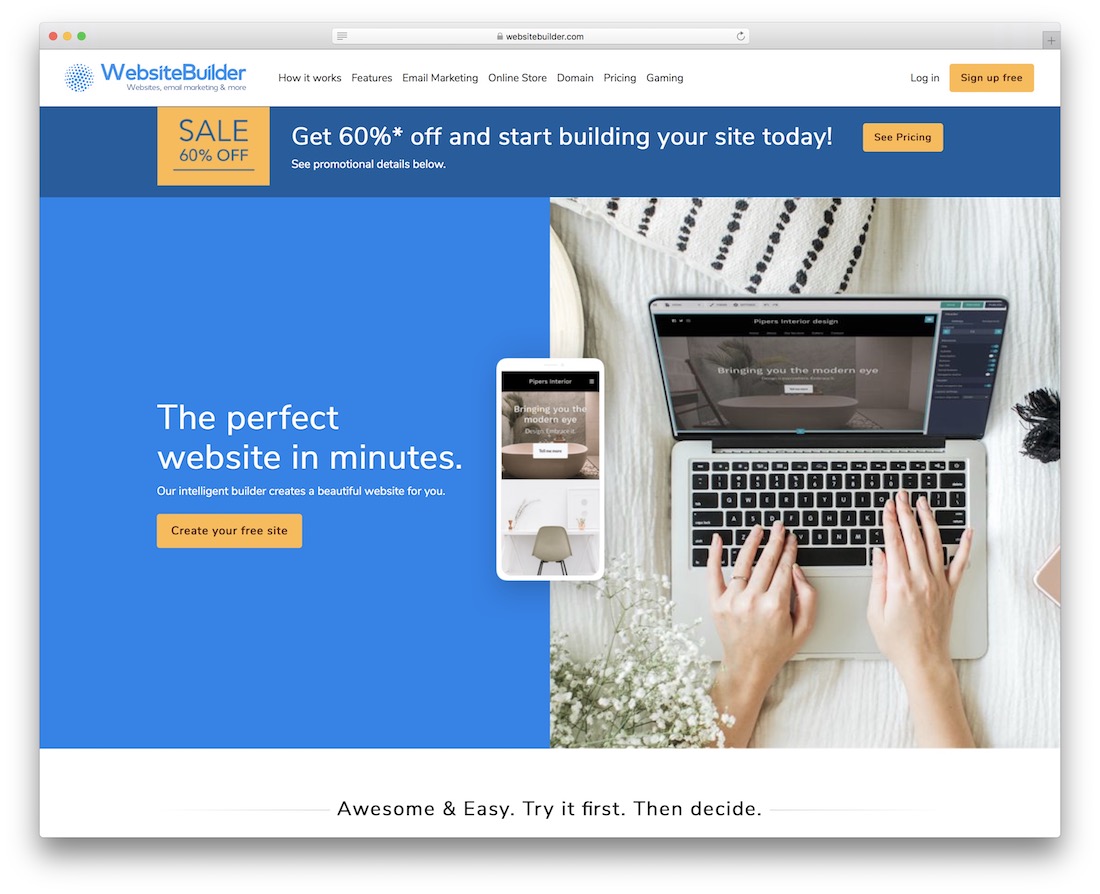"Displayed is an Apple browser window showcasing the Website Builder homepage, identifiable by the characteristic red, yellow, and green circles at the top left corner. The Website Builder logo, a circular icon with multiple dots at the center, is situated in the top left of the webpage. The navigation bar, located centrally at the top, includes tabs for 'How It Works,' 'Features,' 'Email Marketing,' 'Online Store,' 'Domain,' 'Pricing,' and 'Gaming.' On the top right, there is a login area accompanied by a prominent yellow 'Sign Up Free' button.

A highlighted promotion offers a 60% discount, urging users to start building their site today, with details and a 'See Pricing' button available to the right. The main image features an individual working on a laptop, identifiable by their hands—one adorned with a ring—and surrounded by white flowers, all set on a white bedsheet. To the left of this image, the text reads 'The Perfect Website in Minutes,' accompanied by a yellow 'Create Your Free Site' button."